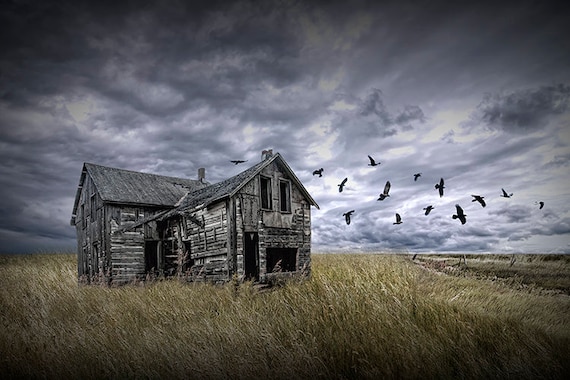In this highly detailed, possibly digitally generated image, an eerie, abandoned two-story wooden house stands alone in the middle of a vast, grassy meadow. The house, grey and blackened with age, appears broken and damaged, with a chimney on top, triangular roofs, vertical long doors, windows, and possibly a fireplace. The surrounding grass is tall and varies in color from green to brown, adding to the sense of desolation. Birds, resembling eagles or ravens, fly in an oddly organized manner around the house. The sky above is filled with dark, stormy clouds, with glimpses of whiteness peeking through, casting an ominous shadow over the entire scene. There are no other man-made objects or mountains in the distance, enhancing the sense of isolation. Despite its photographic quality, the image has an almost surreal perfection that suggests it might be AI-generated.